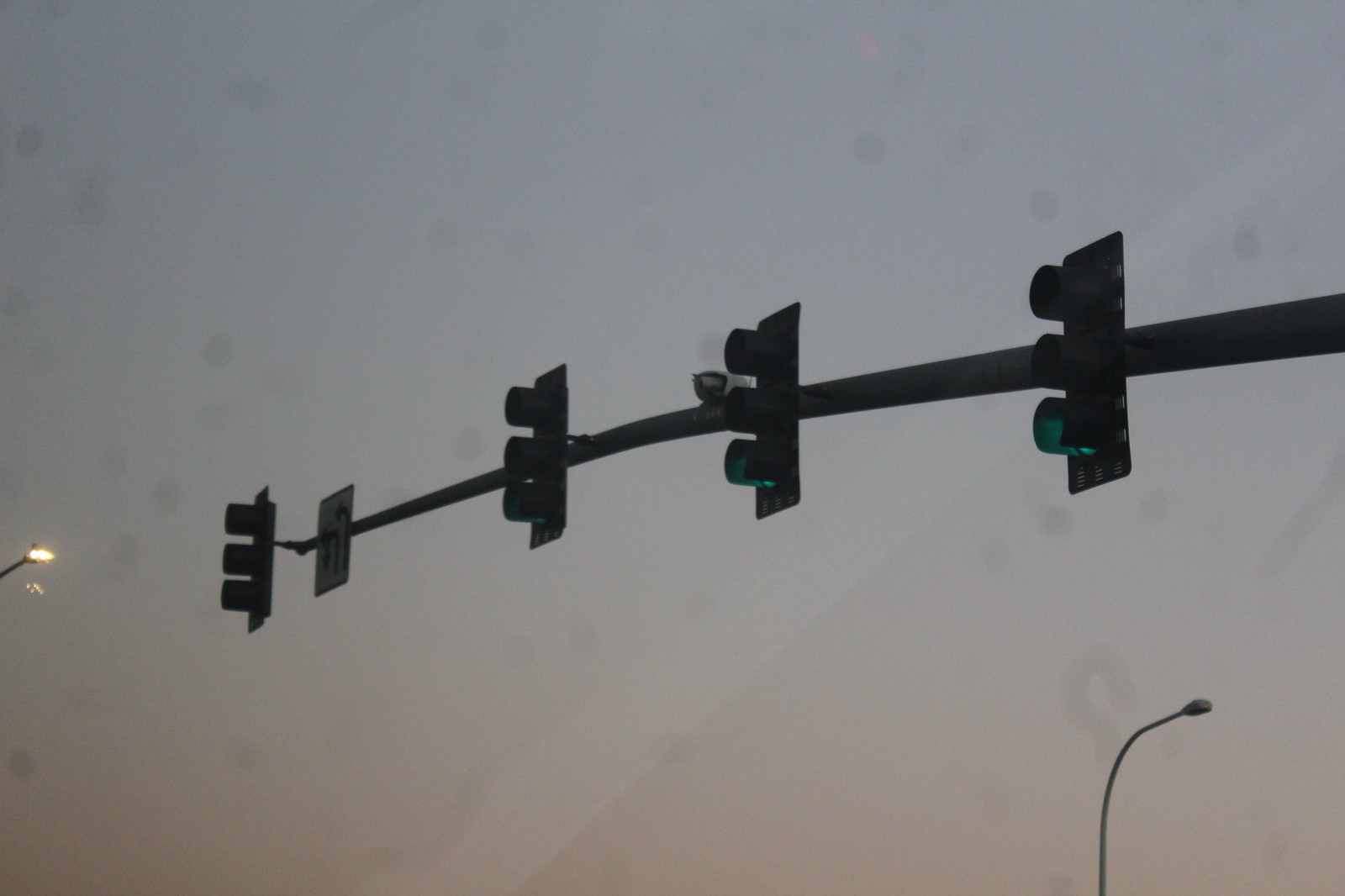In this image, a large horizontal pole extends across the sky, featuring four traffic lights arranged as if overseeing four lanes of traffic. The scene unfolds under a mostly gray and blue sky with cloud cover, suggesting a dusk setting, perhaps after a bout of rain. The two rightmost traffic lights are visibly lit green, while the leftmost lights are out of view from the camera angle. A small, curved streetlight is present at the bottom right of the image, appearing unlit. Additionally, there's a sign indicating that U-turns are permitted for the left lane, and a speed camera seemingly hidden between the second and third traffic lights. The overall photograph captures a dimly lit atmosphere with a silhouette-like presentation of the pole and traffic lights against the backdrop of the dusky sky.